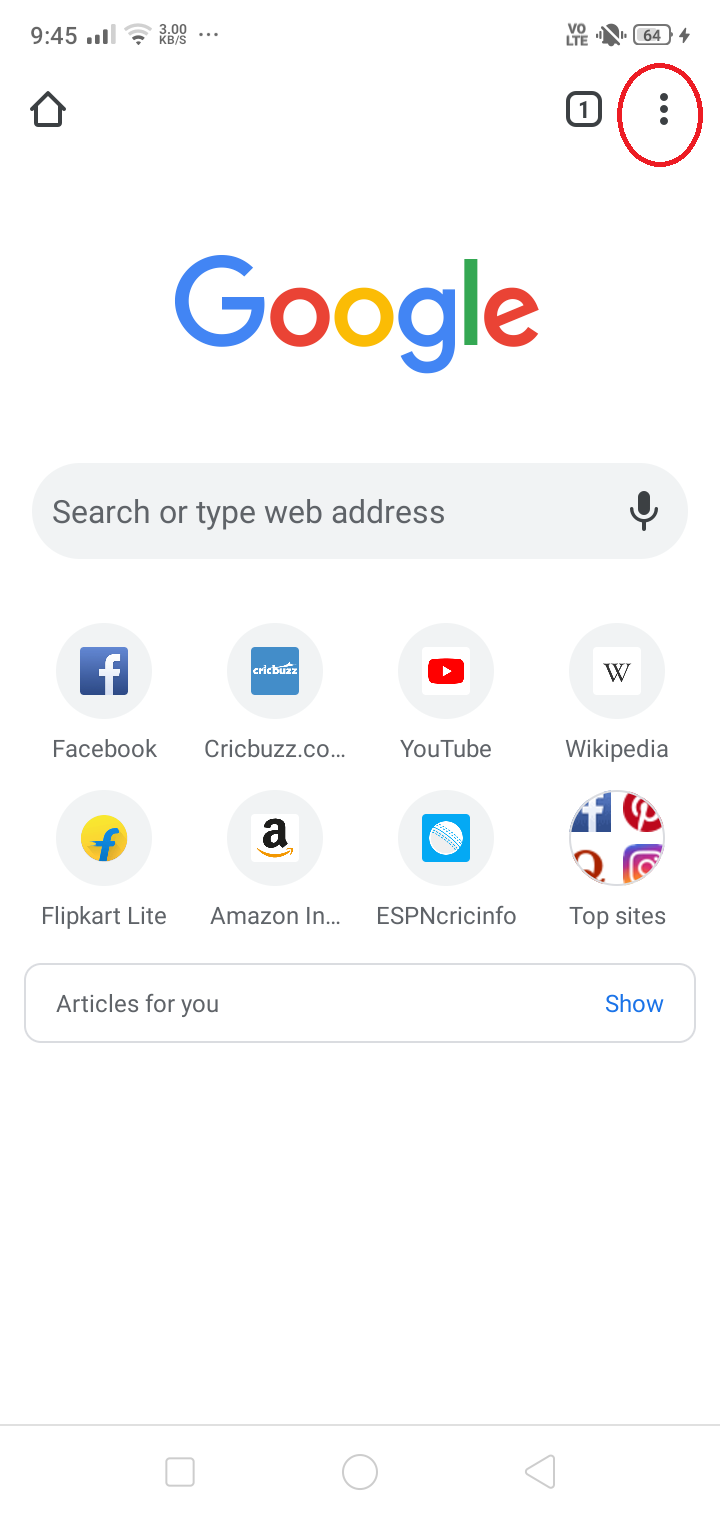An image of a cell phone screen displays various interface elements. The battery life indicator shows approximately three-quarters full, and the current time is 9:45. The network connection signal is moderate. At the bottom of the screen, there's a home button, featuring the Google logo in its distinctive colors: blue, red, yellow, and green. 

In the center, a prominent Google search bar encourages users to "Search or type web address," with a gray background on the right side, featuring a microphone icon for voice input. Below the search bar, several frequently visited websites are listed, including Facebook, chrisbuzz.co, YouTube, Wikipedia, Flipkart Lite, Amazon, ESPN, Crimsonpho, and Top Sites.

The "Top Sites" category includes recognizable icons for Facebook, Pinterest, Instagram, and another familiar site. Further down, the section labeled "Articles for you" is present, accompanied by a blue "Show" button that likely reveals more content when pressed. The overall background of the screen is white, providing a clean and straightforward layout for the listed websites and features.